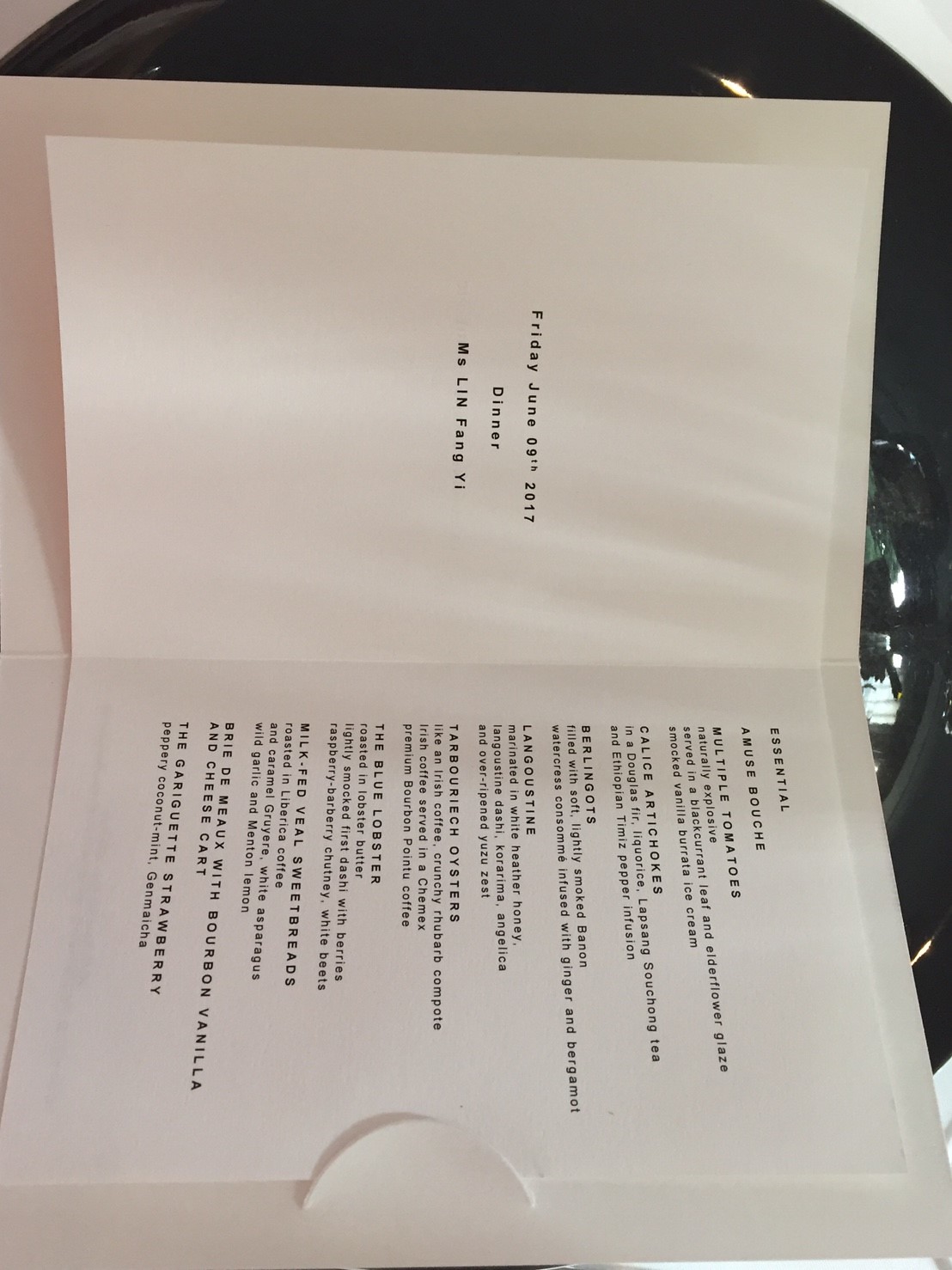This photograph features a minimalist, elegantly folded white piece of paper housed within a white cardstock holder. The holder has a rounded half-circle tab at the lower edge, securing the inner sheet in place. The arrangement suggests that it is a menu or an event schedule. The bifold format of the holder sets the inner sheet sideways, with the top of the text facing right and the bottom facing left.

The white paper, enclosed within the white cardstock frame, is held above a shiny, dark, round metallic surface, possibly a dish, that dominates the background. The metallic surface reflects lighter white areas, indicating its reflective nature. Only the corners of a white tabletop are visible beneath this metallic object.

The menu text is printed in a small, hard-to-read font. On the visible left page, three lines of text can be discerned: the first line reads "Friday, June 9th, 2017," followed by the word "Dinner" in the second line, and finally, a name, "Ma Lin Feng Yee," on the third line. The right page, situated at the bottom, is densely packed with multiple lines of text, listing nine items with descriptive paragraphs and two headers at the top, though the specifics are too small to be legible.